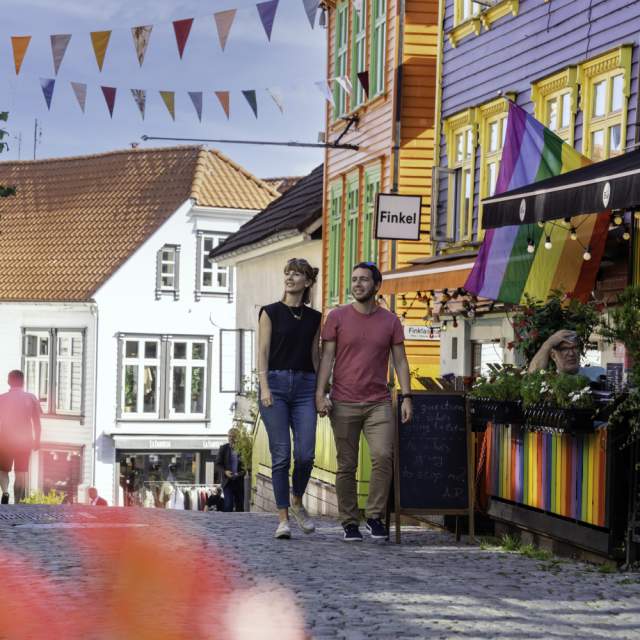In the vibrant photograph, a couple is seen walking hand in hand through a colorful European town, perhaps as tourists enjoying the picturesque scenery. The man is dressed in a red t-shirt, tan slacks, and black sneakers, while the woman wears a sleeveless black top, blue jeans, and white sneakers. Both are smiling and looking off to the left, captivated by something delightful in the distance. They stroll on a charming old cobbled street, with bright, vividly painted buildings lining the path. Prominent is a yellow building with yellow window frames and an adjacent orange building with green window frames. A white building with orange roof tiles stands in the background, enhancing the colorful ambiance. There's a restaurant displaying a rainbow pride flag and possibly a chalkboard for specials, contributing to the festive atmosphere. Between the buildings, strings of multi-colored pennant flags dangle, adding to the town’s lively character. A sign that reads "Finkel" is visible, likely indicating a nearby shop or establishment, reinforcing the bustling, welcoming nature of this enchanting town.